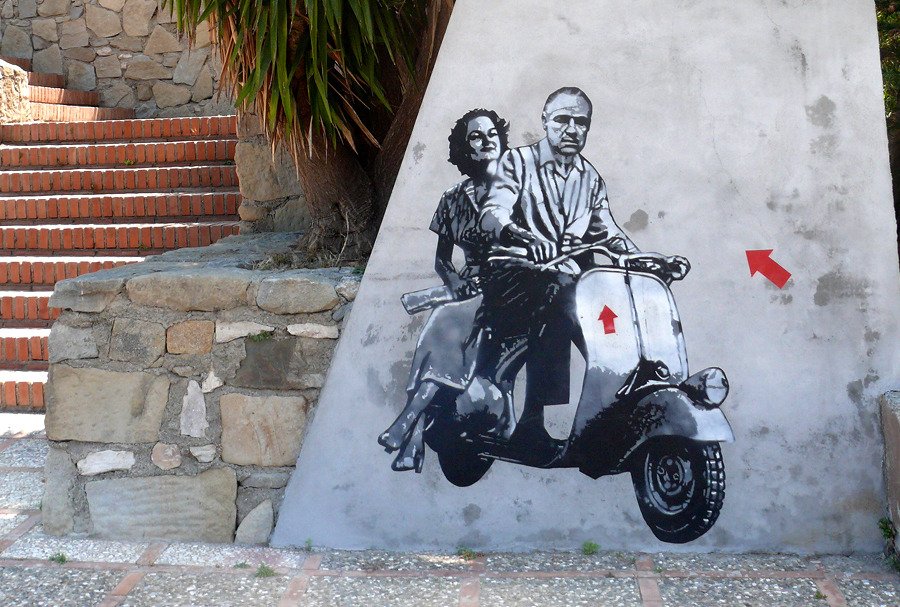The image depicts an outdoor setting dominated by a large concrete retaining wall. On the left side of the scene, there is a set of brick stairs, initially descending four steps from a higher ledge, then leveling out before continuing with another eight steps towards the camera. The steps are bordered by stone-patterned walls. The ground in front of the steps is paved with gray stone.

Centrally positioned on a vast concrete slab, reminiscent of a Banksy stencil style, is a detailed black and white graffiti illustration. The artwork features a man, identifiable as Marlon Brando, and a woman on a vintage Italian-style Vespa scooter. Brando, with a stern expression, is seated astride the scooter, dressed in a white shirt and black pants, and gripping the handlebars. Positioned side-saddle behind him, the woman has short black hair, a short-sleeve shirt, and a short dress. Her legs are draped off to the right with her ankles crossed, and she smiles warmly at Brando.

The scooter has a distinctive shield in front of the handlebars, above which a red arrow points upwards, directing attention to Brando's head. Another red arrow on the right wall points towards the illustration, adding an intriguing detail to the scene. The front wheel exhibits a headlight, enhancing the scooter's authentic portrayal. This captivating and meticulous graffiti invites viewers into a blend of urban architecture and street art.